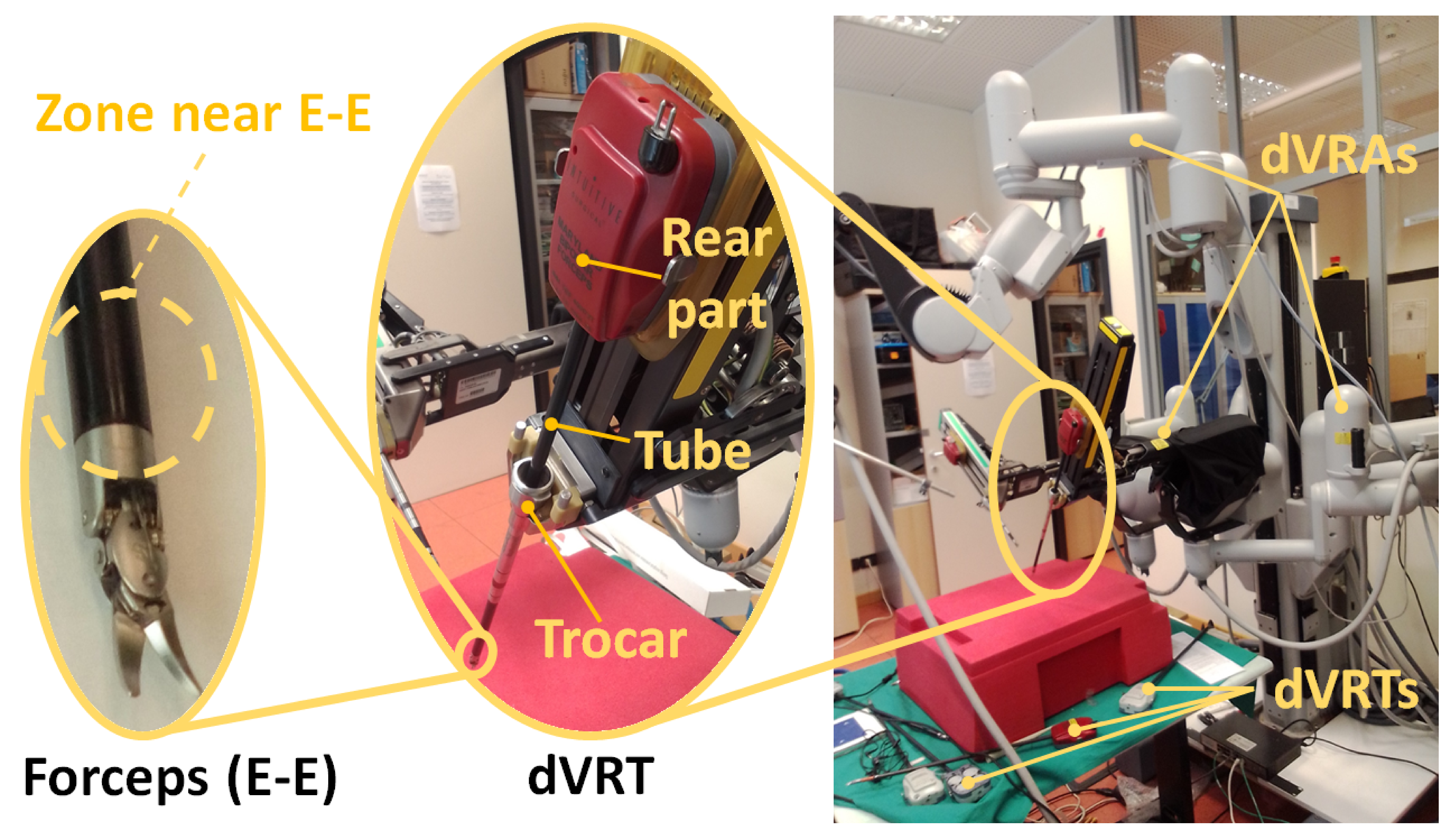This detailed image depicts a complex and intricately labeled piece of mechanical machinery. Various parts are meticulously annotated, primarily using yellow callouts. On the left side of the image, a section titled "zone near EE" is highlighted, extending down to a long cylinder with a black handle and a sharp, pointed end labeled "forceps EE." Adjacent to this is another detailed area, marked by a large red section labeled "rear part," which leads to a tubular component below it labeled "tube," and further down, a piece called "trocar." Beneath this arrangement, the annotation "DVRT" is visible. 

Moving to the right, the image expands to show a larger view of the entire machine. This section has several lines branching out from the word "DVRAS" at the top and "DVRTS" at the bottom, connecting to various machine components. A prominent circle in the center highlights and enlarges specific parts of the machinery for greater clarity. Notably, a red-colored box is placed on a green table on the right side of the image, serving as a vivid point of reference within the photograph.

The combination of detailed annotations and the color-coded callouts provides a comprehensive breakdown of the mechanical components, though the exact nature and function of the machine remain unclear.